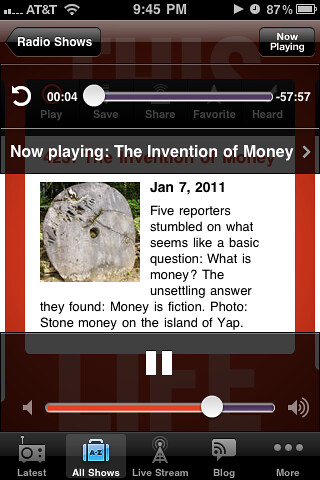This image is a detailed screenshot from an older version of iOS on an iPhone, displaying a podcast interface. At the top of the screen, it shows the AT&T network provider with full service, the time 9:45 PM, and the battery level at 87%. The interface indicates that the user is four seconds into a podcast titled "The Invention of Money," which has a total duration of 57 minutes and 57 seconds. The podcast, dated January 7, 2011, begins with a narration about how five reporters explored the seemingly simple question, "What is money?" and discovered the unsettling notion that money is a fiction, referencing stone money on the island of Yap. The screen also highlights a red volume bar set to more than 50%, with a pause button, and a bottom menu consisting of options labeled Latest, All Shows, Livestream, Blog, and More. The color scheme includes black, gray, white, maroon, red, orange, green, and light blue, making it visually engaging despite the outdated UI design.